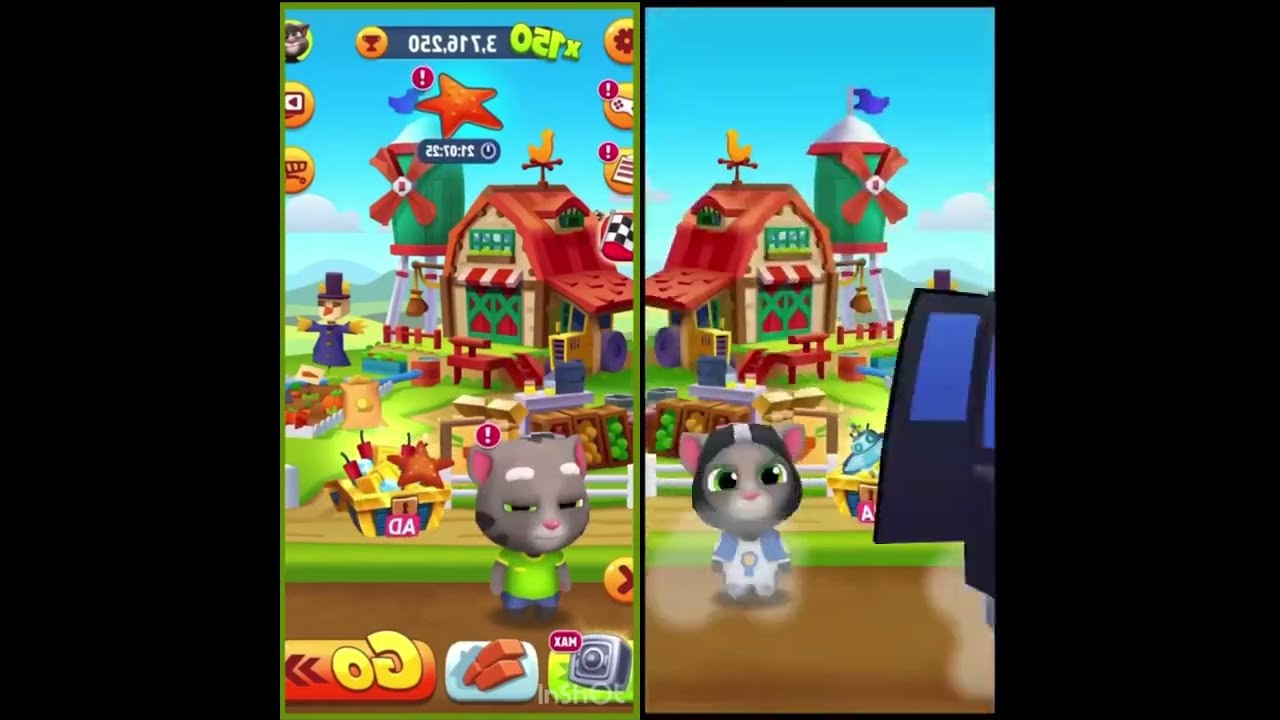The image features two side-by-side screenshots of a colorful, animated children's mobile game set on a farm. Each side is framed by black borders. The left screenshot appears to be reversed, showing all numbers and text backwards. It displays a bright blue sky, a barn, a scarecrow, a timer indicating "150," and a score reading "3,716,250," along with several icons at the bottom. The foreground features a cat character with a rounded body, presumably looking toward the player.

On the right, a similarly designed cat character, this time with a different outfit—wearing a white shirt, purple scarf, and a black hat with a white stripe—stands in front of the farm scene, which includes a windmill, various farm buildings, and agricultural equipment. The cat's ears are perked up, suggesting attentiveness. The farm background is not reversed and appears in its correct orientation. This side of the image also shows elements of a spot-the-difference game, where players might need to compare the two scenes within a split screen to identify subtle differences for points and timed challenges.